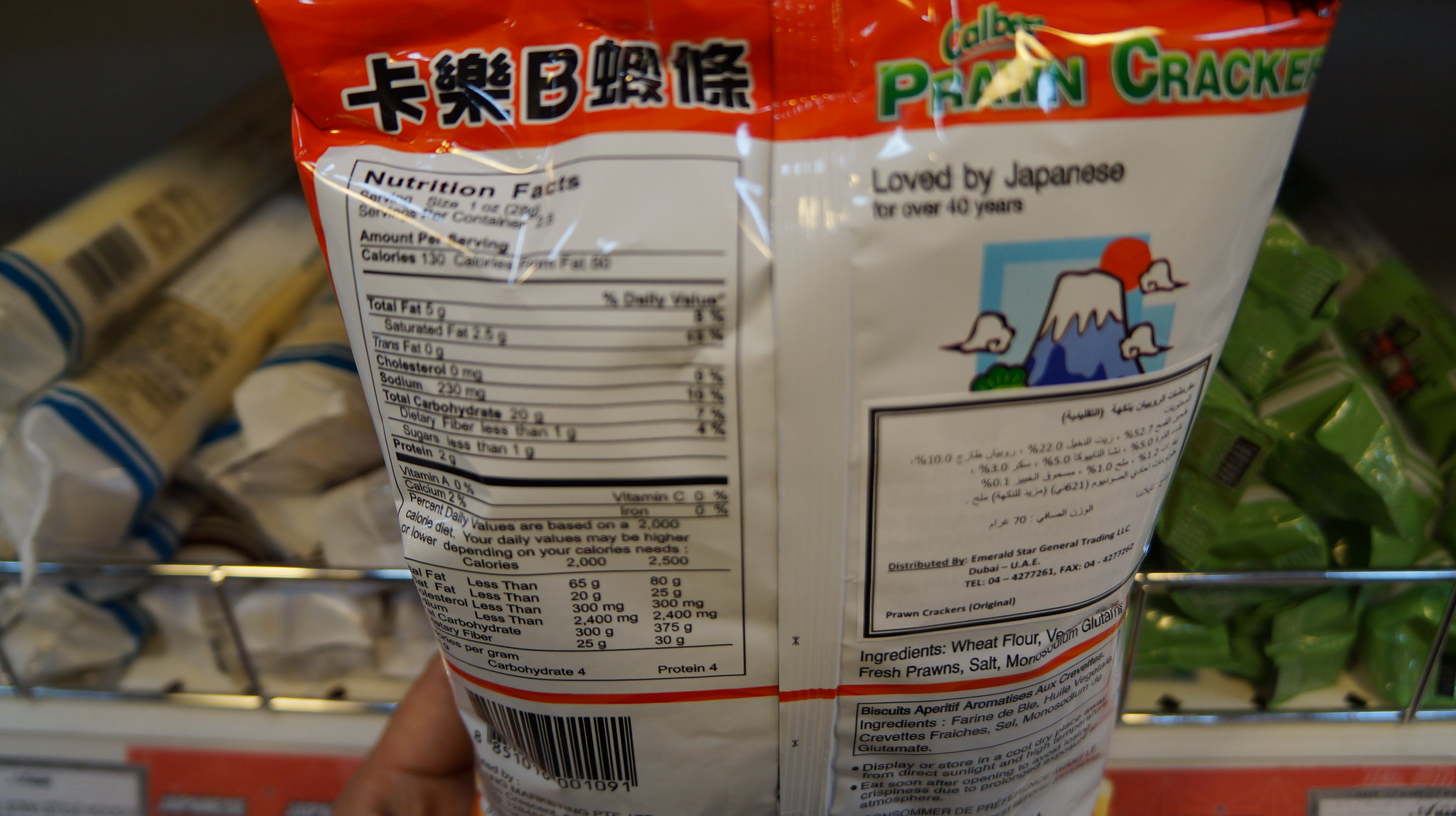The image depicts the back of a package of prawn crackers held up to the camera. The packaging prominently features Asian symbols in the upper left-hand corner. The nutrition facts are printed in English, listing elements such as calories, total fat, saturated fat, trans fat, and cholesterol, though the numbers are slightly out of focus. A hand partially visible on the left side holds the package. On the right side of the packaging, the phrase "Loved by Japanese for Over 40 Years" is written next to a colorful, animated depiction of Mount Fuji. The ingredients listed include wheat flour, fresh prawns, and salt, while the remaining ingredients are obscured. The background suggests the setting is a store, with other packages and items faintly visible.